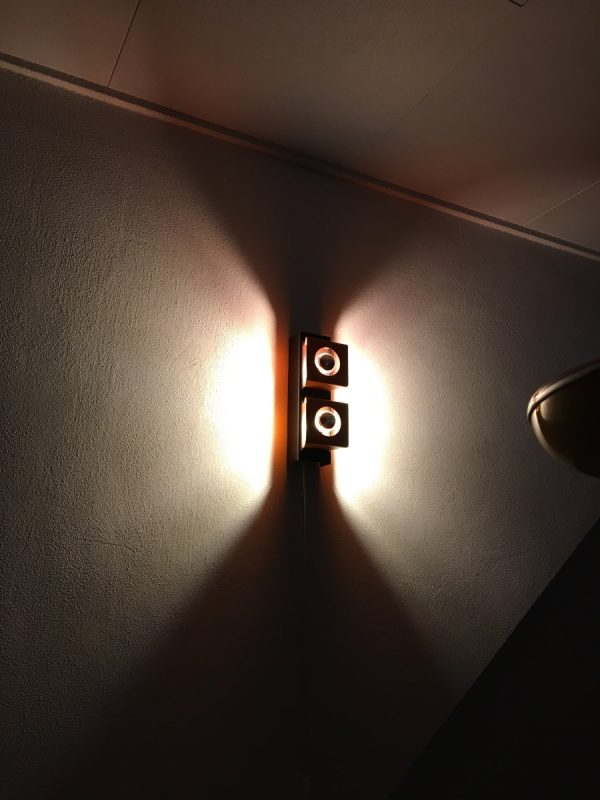The image depicts a dimly lit room or hallway, primarily focused on the upper section of a wall, extending to the ceiling. The space is dark, with the only light emanating from a modern sconce centrally positioned on the wall. The sconce features a sleek, rectangular design composed of two small, black squares with donut-shaped cutouts that emit a brilliant white light. This light, intensified by a clear ring around each square, projects a soft, hourglass-shaped shadow above and below the fixture. Though the exact color of the wall is obscured due to the low lighting—appearing either gray or light blue—the bright illumination from the sconce provides a stark contrast against the otherwise muted background, highlighting the room's minimalistic design.